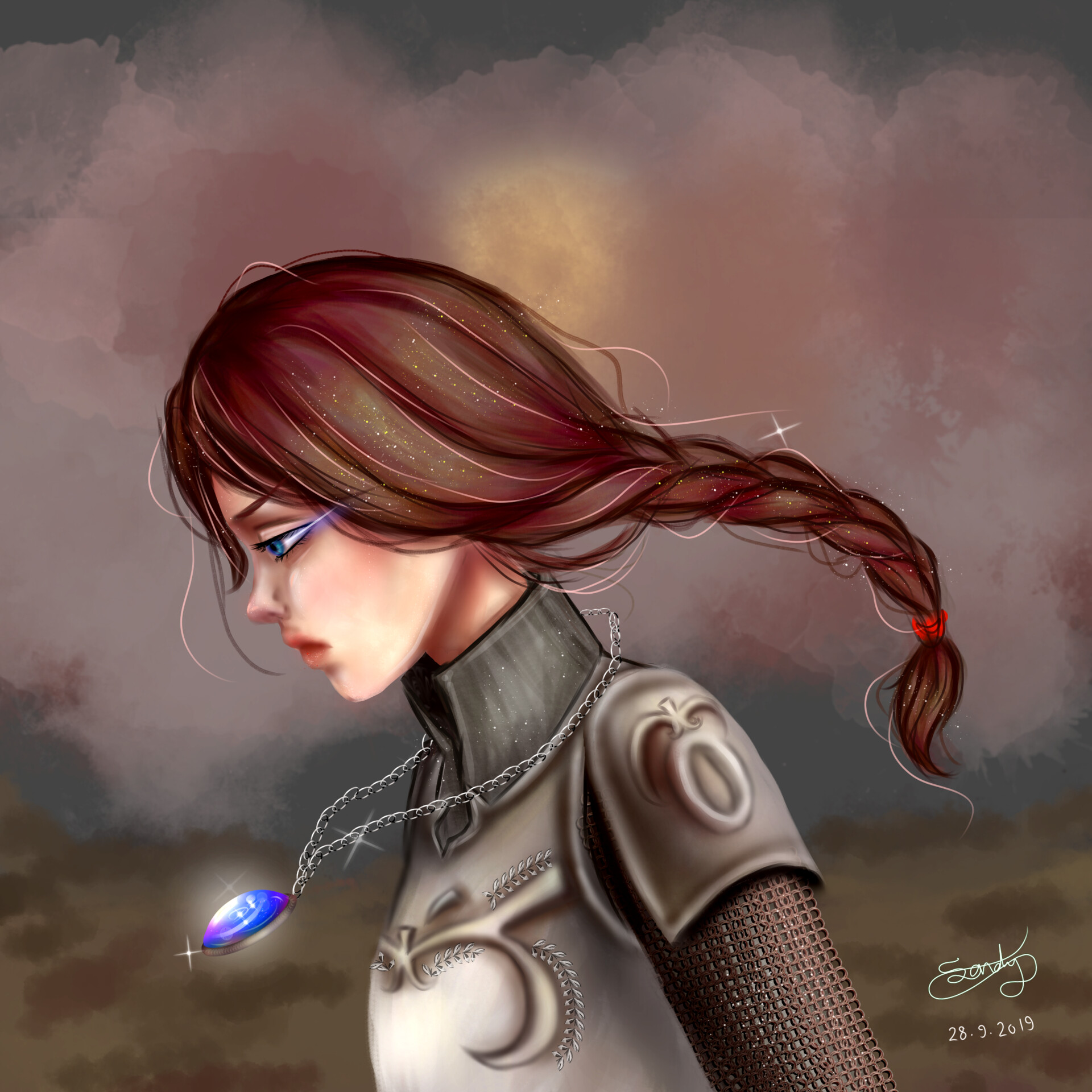The image is an artistic, digitally created profile of a woman with arresting blue eyes and a mix of reddish-brown hair, styled in a floating, braided ponytail secured with a red hair tie. She dons ornate metal armor, adorned with curvy decorations and chain mail on her arm. A silver necklace featuring a giant, glowing blue crystal pendant, reflecting a mixture of purple, blue, and white light, graces her neck. Lavender light emanates from the sides of her eyes, adding a mystical effect. The background is an abstract blend of pink, grayish-blue, and brown hues, blurred to highlight the subject. The illustration is signed "Sandy" and dated September 28, 2019, in the bottom right corner, enhancing its authenticity.